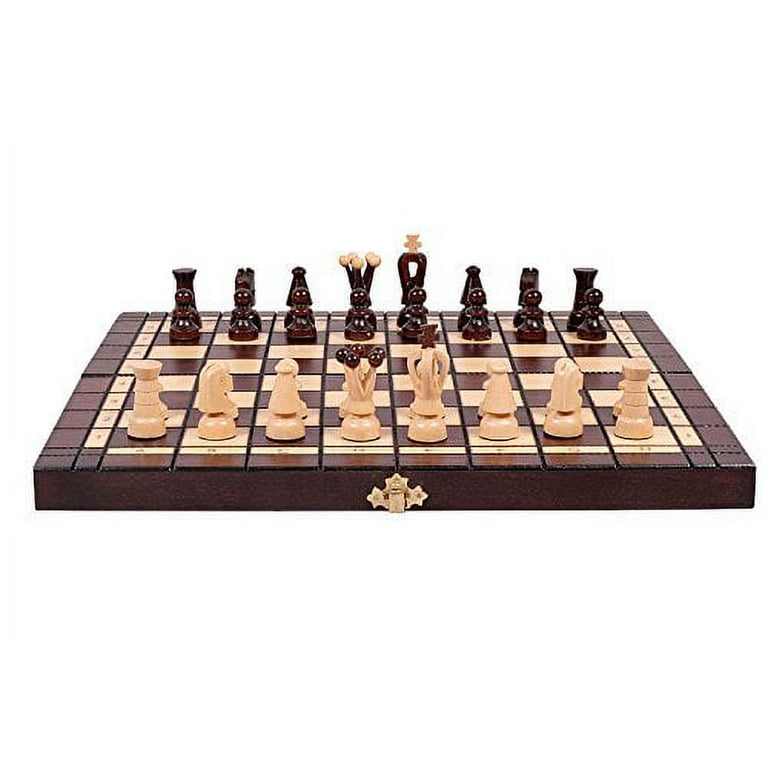The image depicts a color photograph of a chessboard taken from the side, against a stark white background that focuses attention on the board and pieces. The chessboard is crafted from wood, likely painted, with alternating dark and tan squares meticulously divided by black lines. The border of the board is a rich brown wood, enhancing the two-tone aesthetic. Positioned on the near side are lighter tan chess pieces, while the darker wooden pieces line up on the far side. There are eight pieces per side, each uniquely shaped, contributing a comical yet intriguing flair. Among them, some pieces feature distinct characteristics like a cross or balls on their heads. The chess set appears highly decorative, with a gold flowery star design embellishing the side of the board, giving it an ornate look. The setup suggests an engaging match between distinctively styled opponents, portrayed in a manner that almost looks like an artistic advert for the chess set.